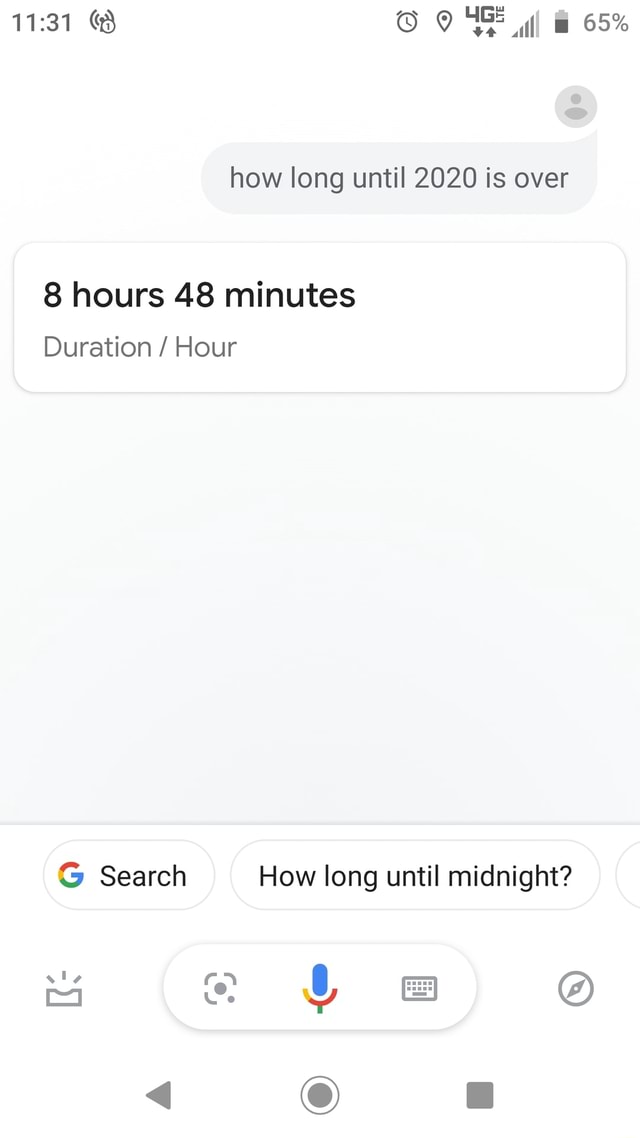This image features a white background with various icons and text distributed across it. Starting from the top left corner, the number "1131" is displayed prominently. Adjacent to it is an icon resembling radio waves, which is often used to depict a microphone sound. To the right of this icon, a grey outline of a clock is visible, followed by a map marker icon.

Continuing along the top, there is a "4G" label with two stars situated underneath it, next to a Wi-Fi signal strength icon. Close to these, a battery icon shows a charge level of 65%.

Below this cluster of icons, on the left side of the image, there is a grey circle containing an image of a person's head and shoulders. Right beneath this circle, in grey text within another grey circle, it states, "how long until 2020 is over.” To the right of these, there is a white box containing the black font text, "8 hours 48 minutes," signifying the time remaining. Below this is the text "duration/hour."

Further down, a grey-shaded box appears, and below this box, on the white background again, a grey circle with the Google logo inside is evident. Next to this, in another grey circle, it reads "how long until midnight."

In the bottom left corner, there is an icon resembling a Kleenex box with three dashes placed above it. Beside this is a grey outline circle with a blue and red microphone icon. Moving to the middle of the image, there is a keyboard icon. Further right, a square grey dot and a grey circle with a line through its side are positioned.

At the very bottom, an array of icons includes a grey triangle pointing to the left, a grey outlined circle with a grey center, and to the far right, a grey box.

This detailed breakdown captures all the elements and visual indicators in the image, providing a comprehensive description of its contents.